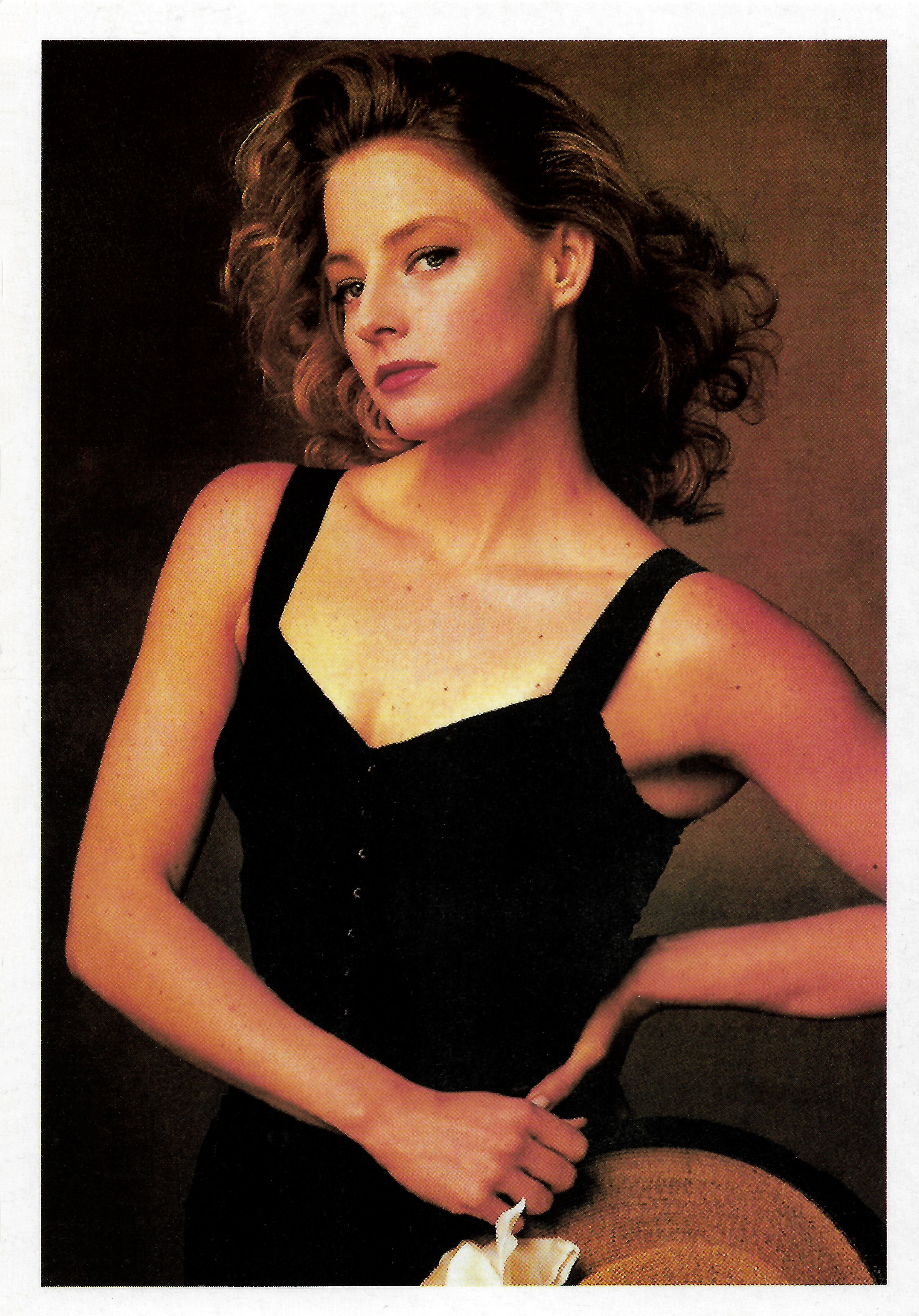The image is a highly detailed portrait, possibly a realistic painting, of a Caucasian woman with light curls and brown hair. She is dressed in a black top with thick straps, featuring buttons down the middle. Her pale skin is adorned with freckles on her chest, and she has striking light blue eyes highlighted with eyeliner. The woman's confidence is palpable; she is not smiling, but her demeanor suggests self-assurance. She has applied red lipstick that accentuates her lips. The background is a gradient of browns, from dark brown at the top left to light brown at the top right. There is a hint of a straw sun hat in the bottom right corner of the image, though it is partially cut off. The photograph, taken indoors without visible natural light, focuses solely on her, making it a classic portrait shot.